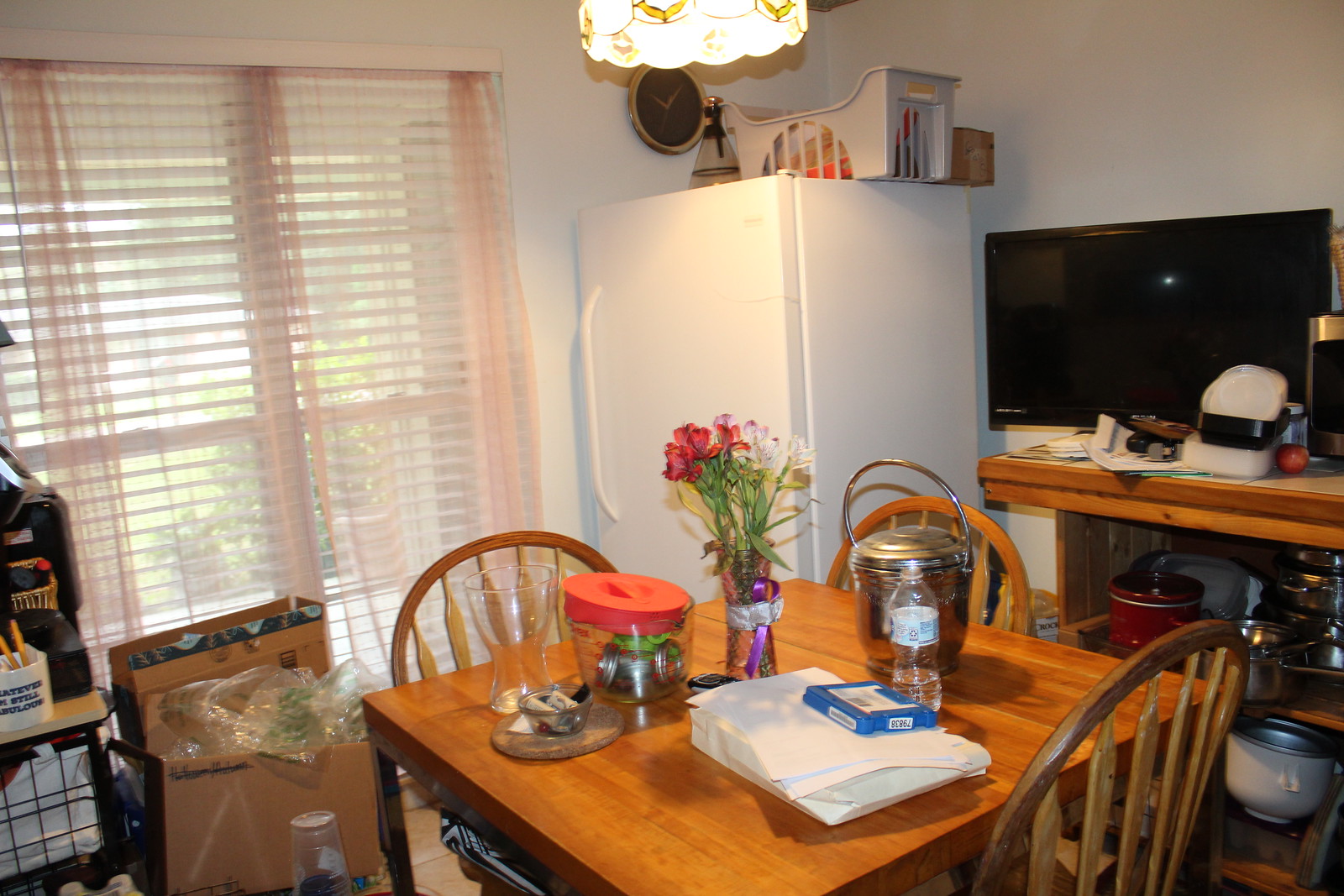A vibrant, colored photograph captures the cozy interior of a kitchen. In the center foreground of the image, a square wooden table is prominently featured, flanked by three wooden-backed chairs. Notably, the left side of the table remains unoccupied, with no chair in sight. Various items adorn the tabletop: a vase brimming with fresh flowers, a large container with a shiny silver handle, a sizeable glass, and an assortment of other miscellaneous objects.

In the background, a small widescreen television sits atop a wooden countertop, which doubles as a storage table with shelving underneath, revealing a collection of pots and pans. To the right of the table, a tall, white, single-door refrigerator is nestled snugly into the corner of the room. The left wall of the kitchen features windows adorned with transparent, pinkish curtains overlaying window blinds, through which a glimpse of verdant shrubs and a well-tended lawn outside can be seen.

Adding to the clutter, two boxes with packaging material spilling out of them are placed in front of the windows. In the far left bottom corner, a small utility table makes an appearance, rounding out the eclectic and homely ambiance of this kitchen space.